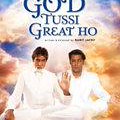This image, though very small, appears to be an album cover with religious themes. It features two men in all-white suits, sitting side by side with their legs crossed. One of the men has his left hand raised, displaying his palm and fingers. Both men have dark brown hair and dark skin. They are set against a sky background filled with clouds of varying colors, including white, gold, blue, and hints of pink, evoking a heavenly, holy feel. The top of the image has text that seems to say, "God to see great hope," although the exact wording is unclear due to the low resolution. The predominant colors in the image are blue, white, and yellow, with some black and possibly brown for the men's hair.